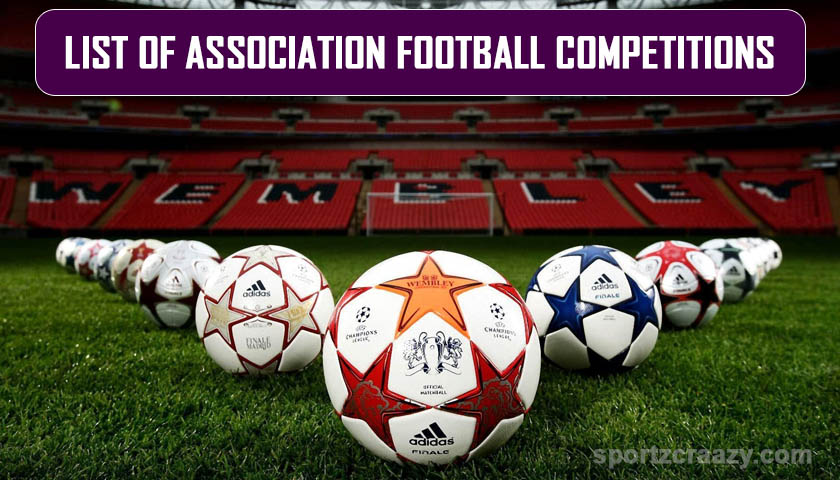The image showcases a vibrant football display on a lush green field. Dominating the foreground is a soccer ball adorned with bold red stars, accompanied by approximately 20 other soccer balls extending in a precise V formation. These balls feature an array of star designs in various colors, including blue, silver, black, and cream. The backdrop reveals red stadium seats spelling out 'Wembley' in white letters, enhancing the scene's athletic ambiance. At the top of the image, white all-caps text in a purple rounded rectangle highlights "List of Association Football Competitions." In the bottom right corner, a subtle watermark from SportsCrazy.com adds authenticity to the vibrant sports setting.